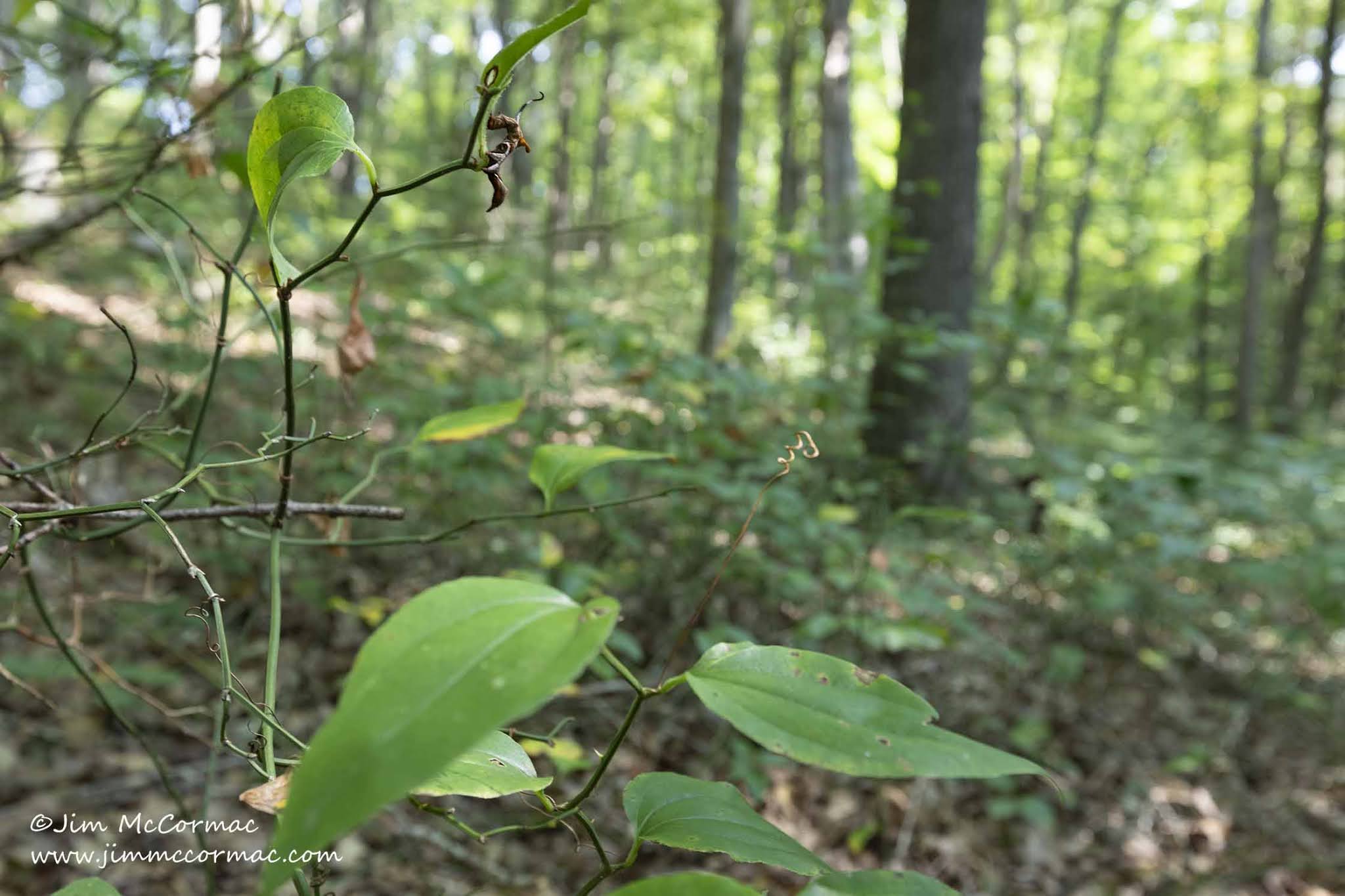This photograph, credited to Jim McCormick at www.jimmcormick.com, captures a lush forest scene on a sunny summer day. The image's primary focus is a close-up of a green plant with a few leaves, some of which show signs of insect activity with small bites and brown spots. This branch, detailed and sharp, stands out against a blurred backdrop of tall trees and dense greenery. The forest setting is teeming with vegetation, visible though indistinct due to the deliberate blurring, which highlights the intricacy of the foreground plant. Twigs and sparse leaves can be seen around the main plant, adding to the natural complexity of this woodland shot. The overall verdant scenery suggests a thriving, vibrant forest environment.